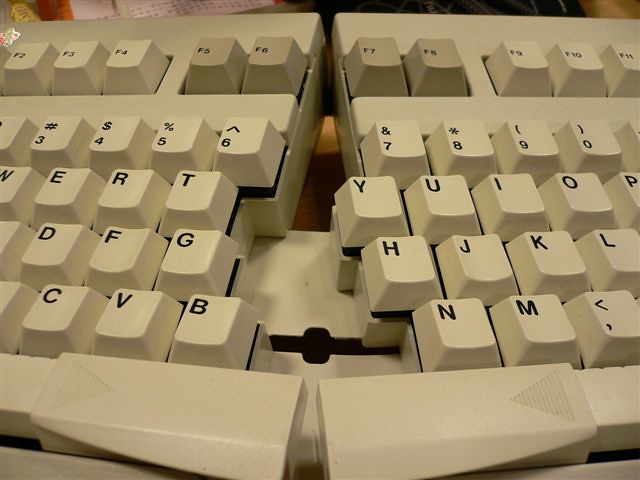This photograph showcases an aged, ergonomic split keyboard with a distinctive yellowed cream color and darker brown raised buttons in the back. The keyboard curves upward at a roughly 10-degree angle, splitting the keys between F6 and F7, the number 6 and 7, T and Y, G and H, B and N, and even the space bar is divided into two separate pieces. Despite its ergonomic design aimed at providing more comfort, the keyboard appears dingy and grimy. Only part of this QWERTY keyboard is visible in the photo, highlighting the left side with keys including W, E, R, T, D, F, G, C, V, B, and the right side featuring keys like Y, U, I, O, H, J, K, L, N, M, and a bracket key, giving an impression of it being used for extensive typing or heavy-duty tasks. This unique layout would likely take some time to adjust to for new users.